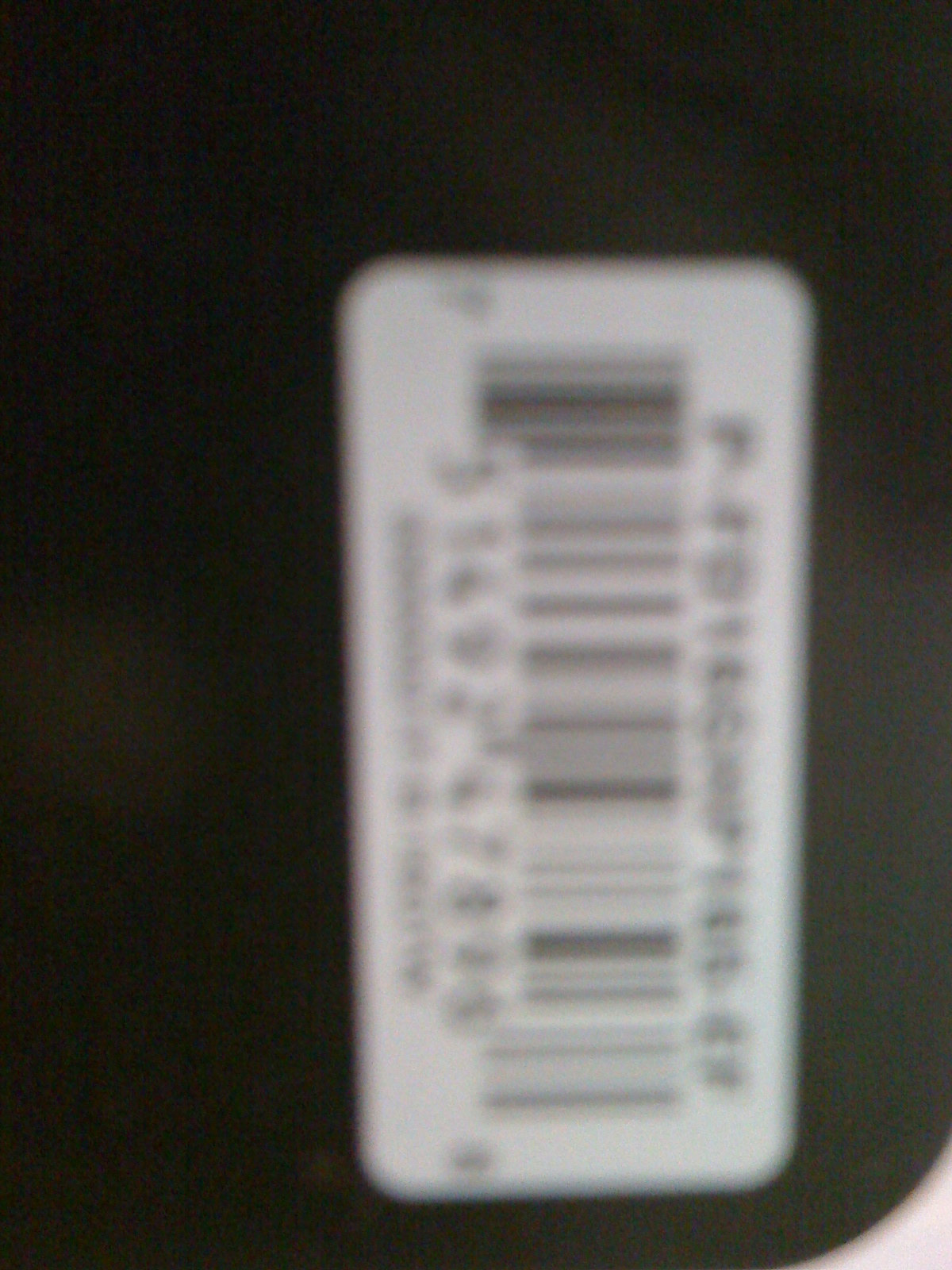This is a very blurry photograph taken by a photographer, capturing a close-up of a barcode sticker affixed to a black object, which comprises the entire background. The barcode is centered and aligned vertically within the image. It is a white label featuring black lines of varying thickness and spacing, characteristic of a typical barcode. Although the image is so blurry that the numbers and letters on the barcode label are illegible, their presence is evident. The background is a light black, and the slightly curved edges of the rectangular barcode give it a distinct shape amid the fuzziness. The photograph’s lack of clarity makes it impossible to determine any specific text, numbers, or the exact nature of the black object to which the barcode is attached.